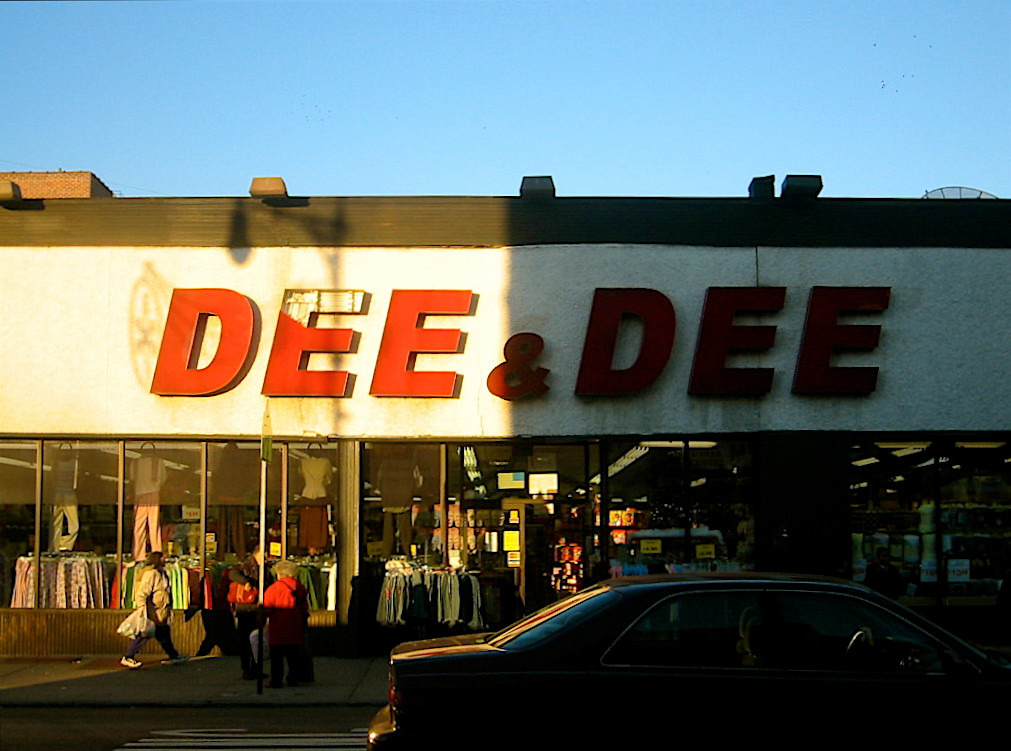The image captures a street scene in front of a vintage clothing store named "D&D" during the late afternoon or early evening, as suggested by the partially lit and shadowed storefront sign. The "D&D" sign, composed of large red letters, shows signs of age and wear, with part of the second "D" missing, revealing the underlying color. Outside the shop, several garments are displayed on racks, accompanied by price signs, hinting at a fall or winter setting due to the nature of the clothing.

In the foreground, three individuals are visible, dressed in long sleeves, jackets, and jeans with sneakers, reinforcing the seasonal atmosphere. The store's interior also features displays of long sleeves and long skirts, contributing to the overall autumnal or wintry context.

Parked in front of the store is a black car, empty but clearly visible. The entire scene is bathed in the soft, golden hues of the setting sun, casting long shadows and highlighting the nostalgic charm of the old clothing shop.